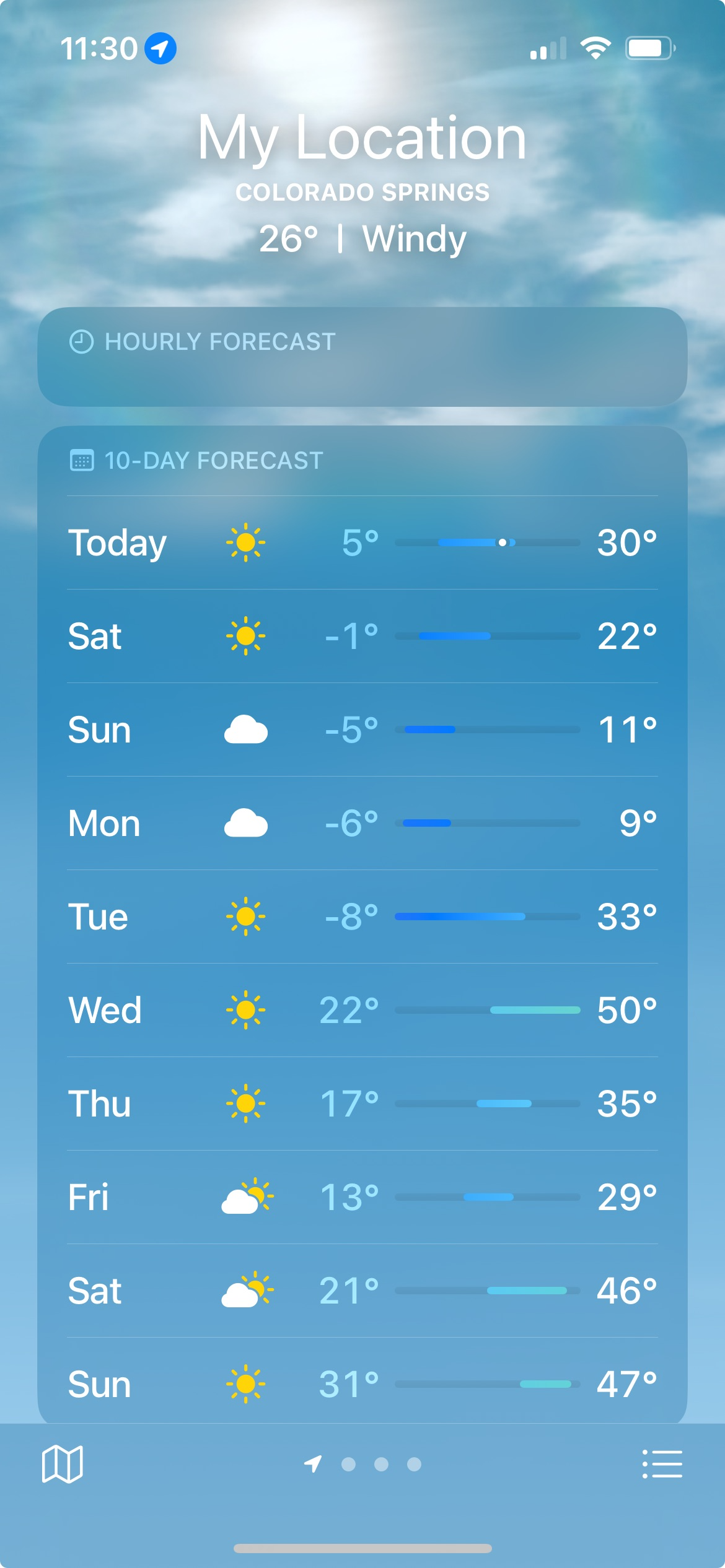Screenshot of a smartphone displaying a weather application. The background is a clear, bright blue sky with scattered clouds, with a prominent white glow in the center, representing the sun. The time shown on the top left is 11:30, and the phone's battery is nearly full, volume is at maximum, but it only has two bars of signal strength. The location is set to Colorado Springs, where the current temperature is 26 degrees Fahrenheit with windy conditions. The visual also includes a 10-day forecast feature, with today being Sunday, predicting a high of 30 degrees and sunny weather. Throughout the next week, temperatures fluctuate, with next Sunday showing a low of 31 degrees and a high of 47 degrees. The interface is clean and predominantly sky blue, with an option to switch to an hourly forecast available at the top of the screen.